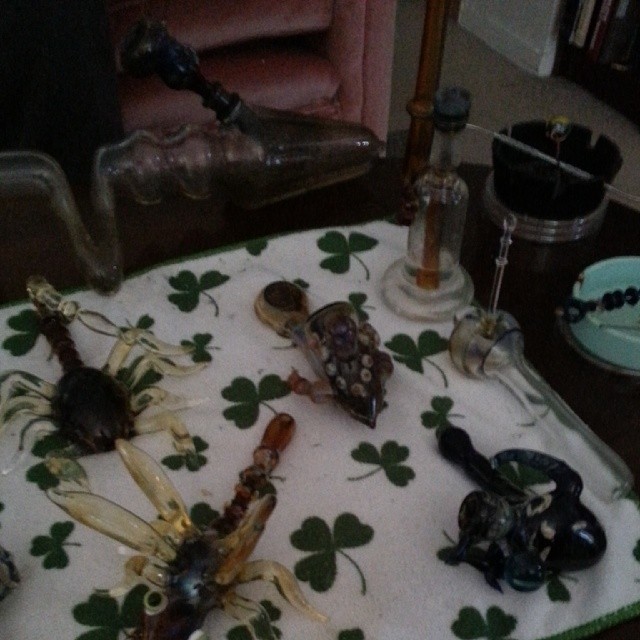The photograph depicts a dark indoor scene of a dark wood table covered with a white tablecloth adorned with green shamrock clovers. The image is notably dim, making it challenging to discern finer details. Spread across the table are various glass figurines that double as smoking devices, possibly intended for substances like marijuana or tobacco. Noteworthy figurines include a glass dragonfly perched atop a pipe in the foreground left, a crouched frog to the right, and a scorpion in the upper left corner. Additional smoking paraphernalia, such as ashtrays, are visible, with a black one on the right side and an aqua-colored vessel next to it. The surrounding environment is dimly lit, featuring a pinkish background on the left, a gray floor, and a white wall with a black border on the right.